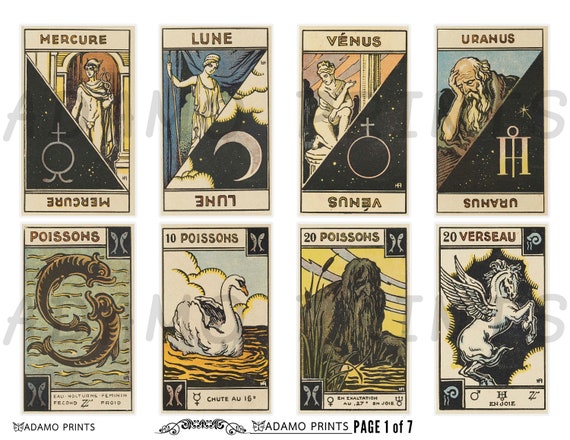This image features a collection of eight vintage-style digital prints, each resembling a card. These cards showcase celestial and mythological themes, likely depicting gods or planets, arranged in a rectangular layout. At the top left, there's a card labeled "Mercure," adorned with a statue and an associated Mercury symbol, with the word appearing both normally and upside down. Next to it is a card titled "Lune," which features a loon and a moon symbol. Following are cards for "Venus" and "Uranus," each with respective statues and symbols—a statue with the Venus symbol and an old man holding his head for Uranus.

Moving to the bottom row, the first card is labeled "Poisons" and depicts two fish. The next two cards also bear the "Poisons" label but feature differing images—a duck and a swamp-like figure, respectively. The final card is labeled "Verseau" and portrays a unicorn with wings. Each card contains a mirrored version of the text, much like traditional playing cards. The prints are in shades of brown, green, and yellow, giving them a classic, aged aesthetic. At the bottom of the image, there is text reading "Adamo Prints, page one of seven," indicating the print series, alongside a watermark "Adamo Prints" across the images.